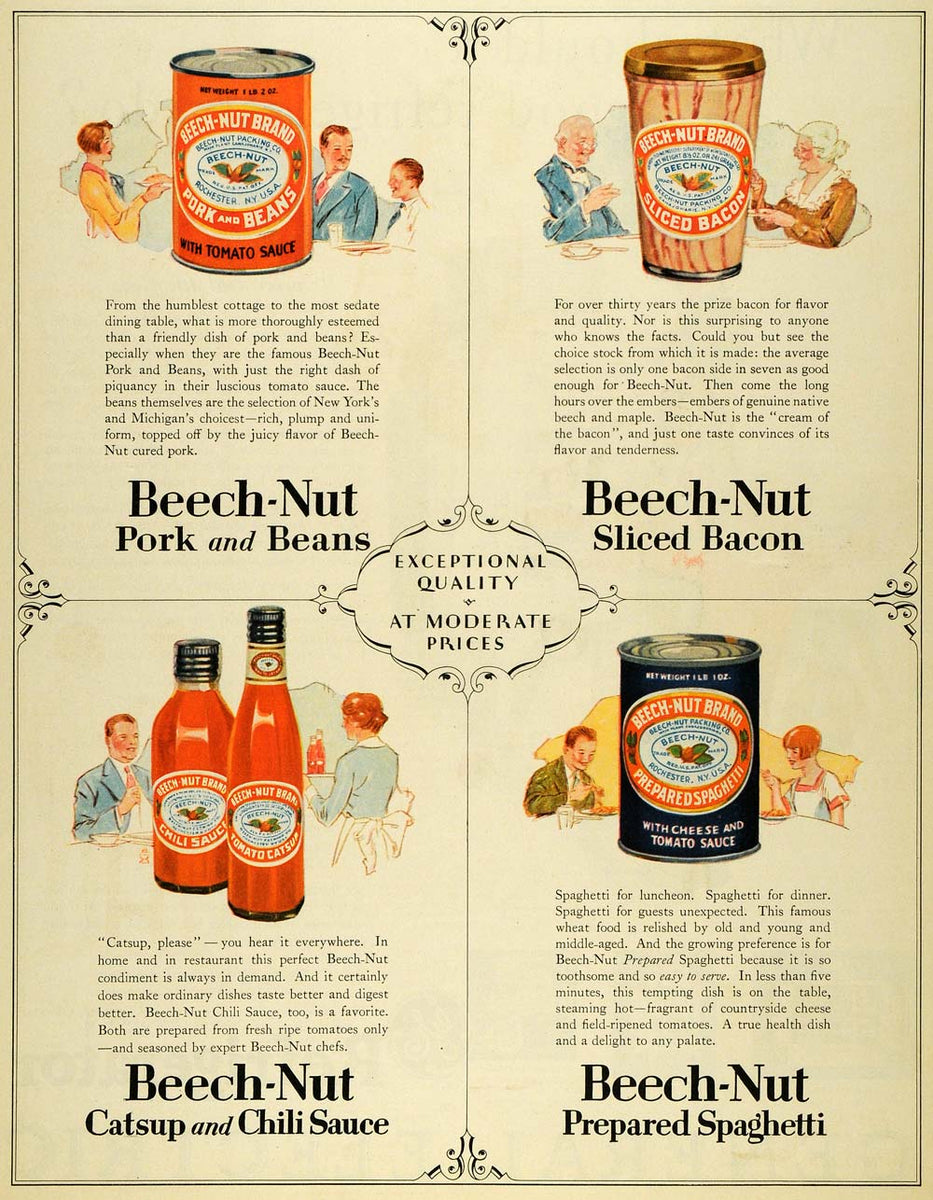The image is a vintage advertisement from the 1950s for Beech Nut products, neatly divided into four main sections. Dominating the center is an ornate oval frame with the Beech Nut logo and the prominent tagline "Exceptional Quality at Moderate Prices." 

In the top left section, the ad showcases a vibrant orange can of Beech Nut Brand Pork and Beans with Tomato Sauce. The heading "Beech Nut Pork and Beans" is boldly displayed below a paragraph of descriptive text. A man in a blue suit and red tie gazes warmly at a child in a white shirt and black tie, evoking a sense of family and tradition.

The upper right quadrant highlights Beech Nut Sliced Bacon, presented in an eye-catching tin. Directly below, the label "Beech Nut Sliced Bacon" is underscored by a detailed paragraph. In the vicinity, an elderly woman and an old man illustrate the timeless appeal of the product.

In the bottom left section, two bottles of Beech Nut Catsup and Chili Sauce are featured, with the labels "Beech Nut Catsup" and "Beech Nut Chili Sauce" neatly positioned underneath. The bottle on the left is notably shorter and wider, while an adjacent photograph shows a couple sitting at a table, enjoying their meal.

Finally, the bottom right quadrant presents a black can of Beech Nut Prepared Spaghetti with Cheese and Tomato Sauce. The text "Beech Nut Prepared Spaghetti" lies beneath another descriptive paragraph. To the sides of the can, a man and woman are depicted savoring their spaghetti, reinforcing the product’s appeal.

Overall, the advertisement blends visual elements of people enjoying meals with detailed product information, all underscored by the promise of exceptional quality at moderate prices.